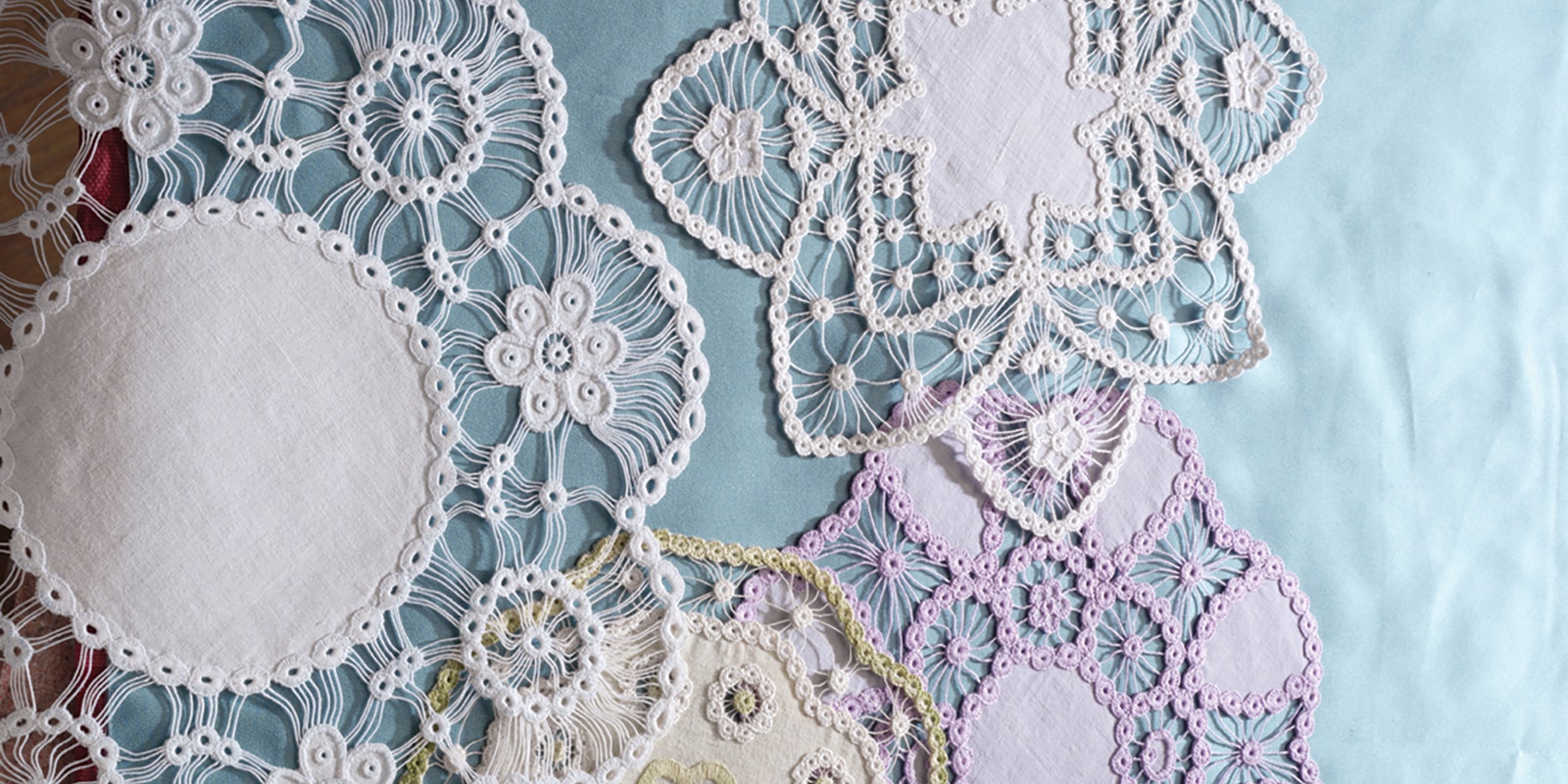This is a highly detailed horizontal rectangular photograph showcasing vintage doilies crafted with intricate, crisscross patterns. The doilies are arranged on a predominantly light baby blue surface that covers most of the background, with hints of reddish-brown possibly representing the edge of a table on the left side. There are a total of four distinct doilies visible in the image: a large, partially visible white doily with a solid center and a lacy floral border; below it, a delicate cream-colored doily with a thick, textured rope-like pattern and an amber border featuring spaced, delicate tentacles and circular designs; further down, a pink doily, appearing almost lavender, with solid areas and an elegant, wavy oval shape only partially visible, displaying a unique top half; and finally, another white doily with a striking eight-point snowflake design, with rounded points converging towards a star-studded center resembling a flower with petal-like extensions. The doilies form a beautiful array of circular, star-shaped, and half-spherical patterns, each showcasing masterful craftsmanship.